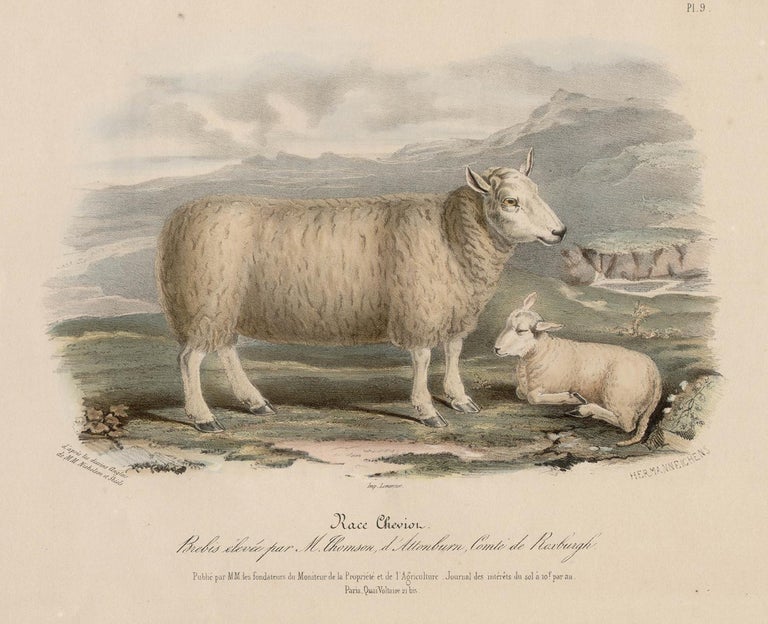This is an aged, vertical rectangular page from a book, identified as PL.9 in the upper right corner. The background of the page is a light tan color that appears weathered. Dominating the center of the image is an illustration of a sheep, facing towards the right. The sheep has a woolly coat, primarily white with some gray and brown tones and black flecks. Its legs are white, and it stands in a grassy, rocky field that extends into a mountainous landscape sketched in shades of brown and gray. 

Lying curled up at the foot of the standing sheep is a lamb, smaller and less fluffy, with solid white fleece and closed eyes. In the background, there appears to be cloudy skies and possibly some water in one area, enhancing the pastoral scene.

At the bottom of the image, in cursive script not written in English, is the text "Race Chevillon," accompanied by additional small, indecipherable print.